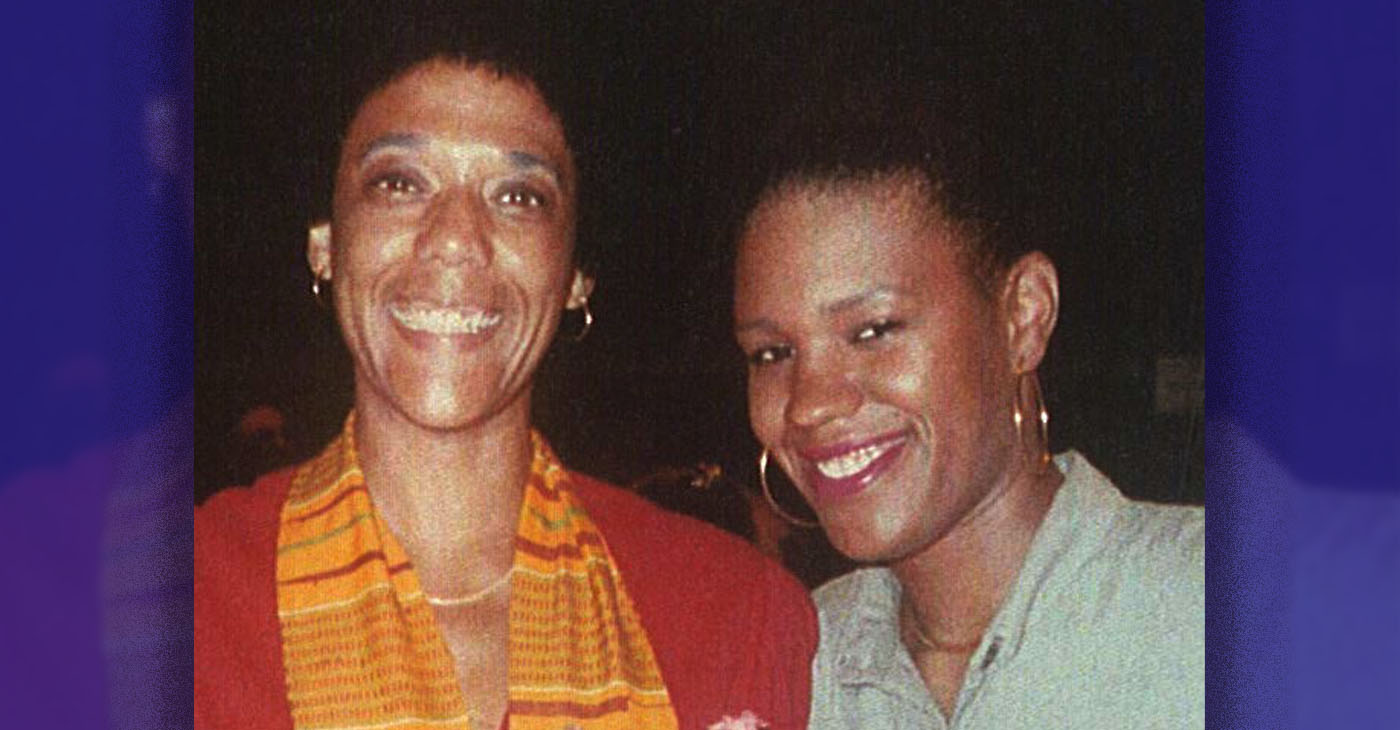In an old-style photo resembling a 1970s snapshot, two African-American women stand against a dark black background, both smiling warmly. The image features a semi-transparent navy blue border, allowing faint visibility of their attire. The woman on the left is slightly taller, with short black hair, thin black eyebrows, and brown eyes. She showcases a lovely, open-mouthed smile despite some imperfections in her teeth, accentuated by light red lipstick. She has mouth lines and adorns gold hoop earrings—larger in size—along with a gold herringbone necklace. Her outfit consists of an orange scarf with white and red stripes interspersed with dotted patterns, over a red sweater. Beside her, the slightly shorter woman also has her hair up, thin eyebrows, and wears a striking red lipstick. She, too, is adorned with gold hoop earrings, albeit somewhat smaller, and a gold necklace. Her clothing features a white shirt under a blue-grey blouse. Both women exude a sense of happiness and are captured looking directly at the camera, encapsulating the charm of a bygone era.